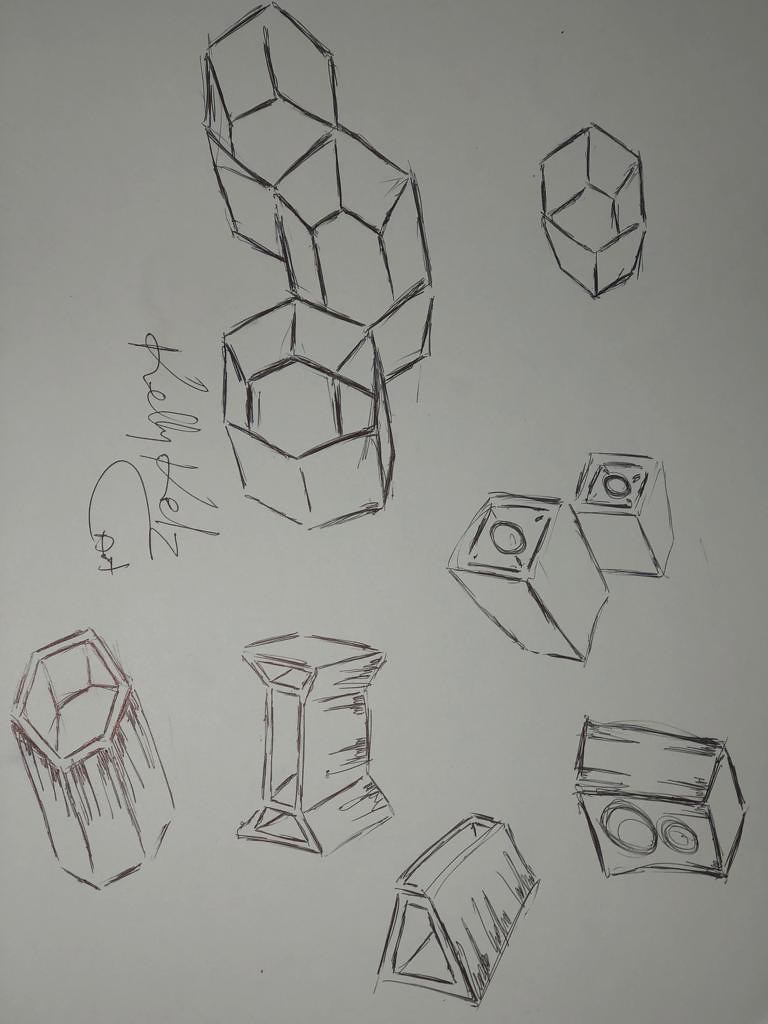This vertical, portrait-style pencil sketch on a white sheet of paper features an array of geometric shapes evenly spread across the page. Signed by Kelly Keltz in the bottom left corner, the drawing consists of several 3D cubes, including a cluster of three at the top center and a separate cube off to the right. Below this, a distinct hollow triangular shape is found in the bottom right. The sketch also includes a singular square and a square box with circles on the right side, as well as additional cube-like and rectangular shapes positioned throughout the middle. The simplistic yet detailed drawing, entirely in tones of grey, is reminiscent of a doodle, potentially by a young artist around twelve years old.